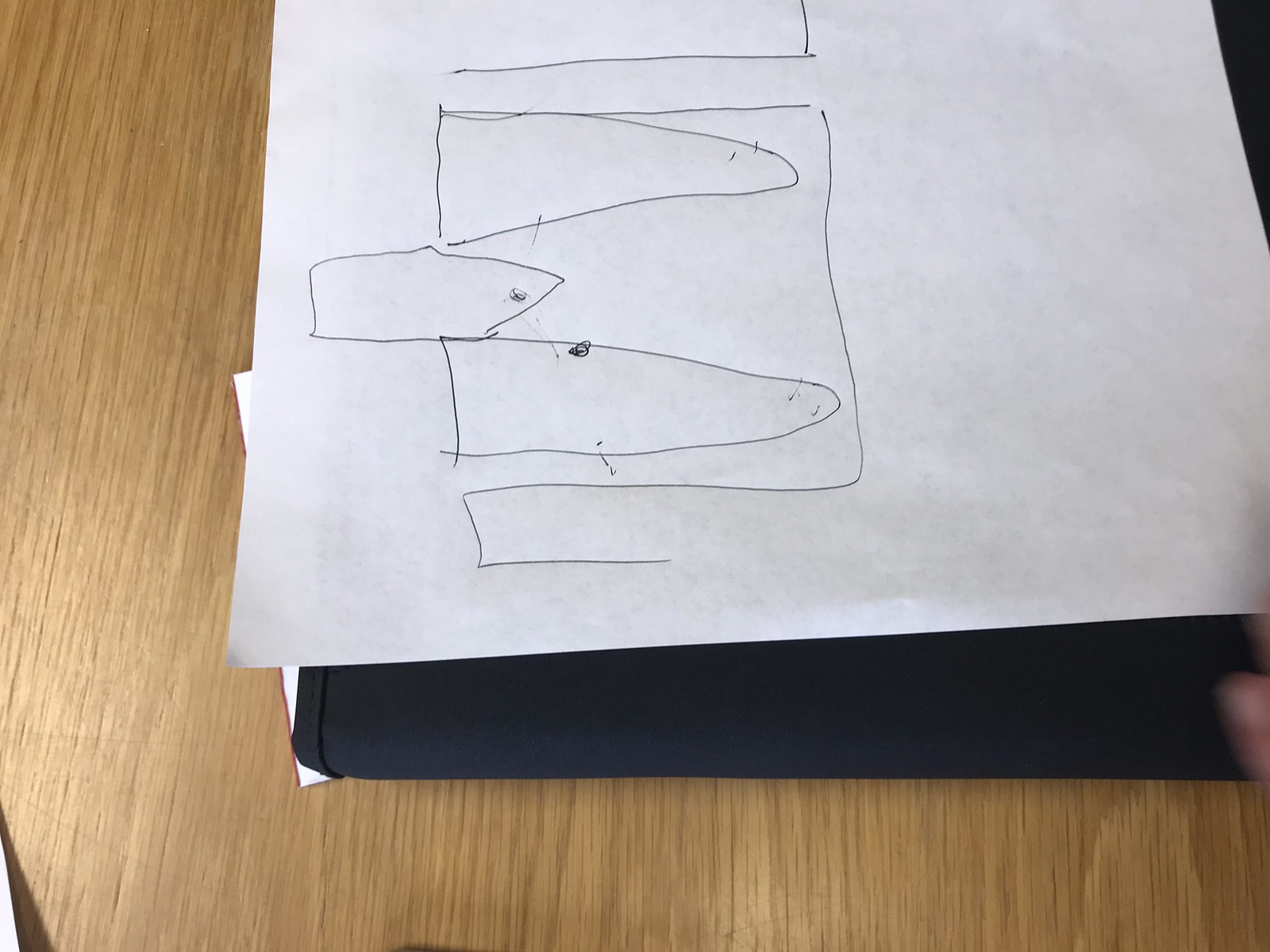The image features a thin sheet of white paper placed atop a black document folder crafted from canvas-like material. This folder is resting on a laminated surface that mimics light brown wood. On the right side of the paper, a thumb or finger, appearing blurry as if in motion, is either holding or touching it.

The paper has been drawn on with what appears to be a black biro pen, discernable by the smudged ink. Dominating the left side of the paper is a large, tall, and thin square containing two mountain-like shapes pointing to the right. Below and outside this square, there is a tall house with a square base and a triangular roof positioned beneath the two mountain shapes. The drawing exudes an abstract, sketch-like quality, with the main elements being the geometric mountains and the singular house.